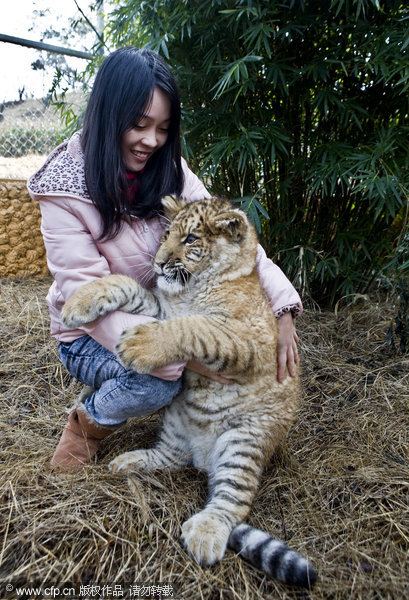In this detailed photograph, a woman with dark black hair, estimated to be in her twenties, is squatting down and cradling a baby tiger cub in her arms. The woman is dressed in a pink coat with a leopard print hood, which is down, blue jeans, and brown Ugg boots. Her expression is one of affection as she smiles at the tiger cub, which has distinctive stripes on its legs and tail, indicating its tiger species despite its initially lion-like coloring.

The setting appears to be an enclosure, likely within a zoo or wild animal compound in China, as indicated by the text "www.cfp.cn" and accompanying Chinese characters visible in the image. The backdrop features overcast skies, green plants, and a fence to the left. The ground beneath them is covered in straw. The woman and tiger cub are centrally positioned, with the cub sitting on the straw and facing towards the left of the image, while the woman is oriented slightly to the right. The overall color palette includes pale yellow, brown, white, green, tan, beige, black, light pink, and a tannish brown color.